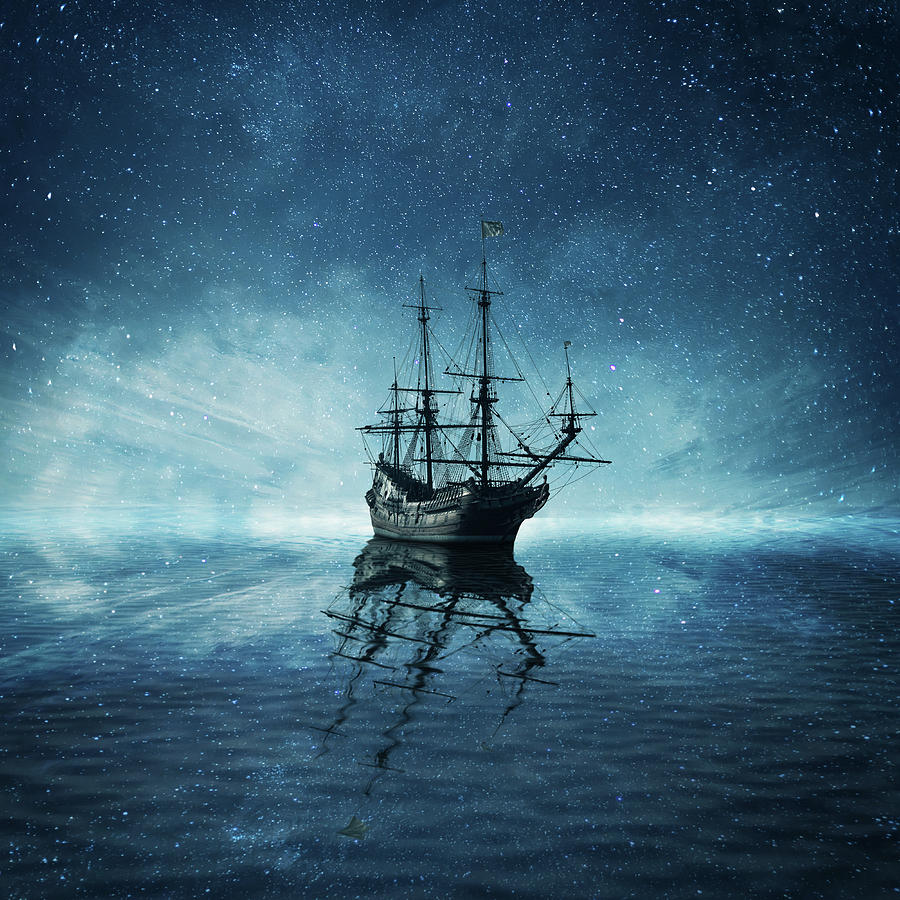The image showcases a mesmerizing, magical night scene featuring an old-timey wooden ship, reminiscent of a pirate vessel, with its four tall masts standing prominently against a dark, star-studded sky. One of the masts is adorned with a white flag. The ocean mirrors the sky so perfectly that it's challenging to discern where the horizon lies. The water around the ship ripples gently, creating a sense of movement, though the ship seems almost ethereal, as if floating or moored for the night. An enchanting bright mist illuminates the ship from behind, enhancing its hauntingly beautiful reflection in the water. The entire scene exudes a serene yet eerie ambiance, with no visible crew, amplifying the timeless and solitary presence of the vessel.